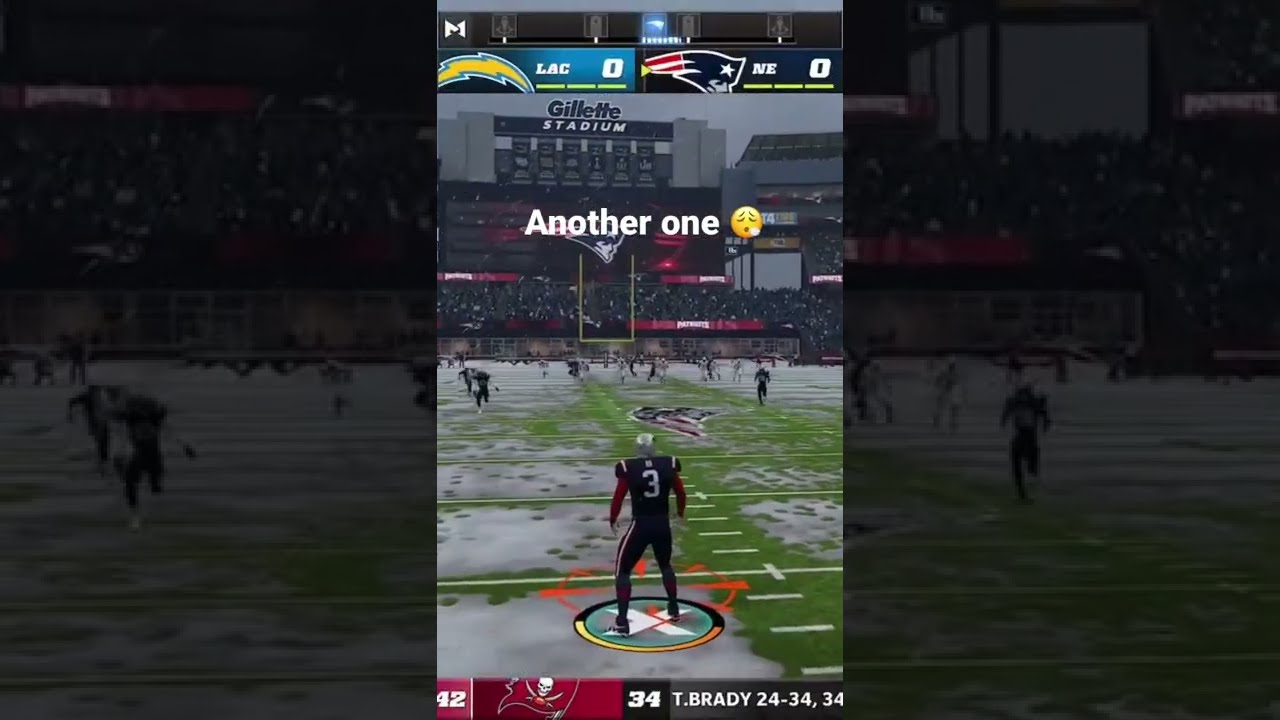This image captures a detailed scene from the Madden video game, specifically a still frame that appears to have been photographed from a phone. The scene is set in a snow-covered Gillette Stadium, home of the New England Patriots. The focal point is a New England Patriots player, number 3, dressed in a dark blue jersey and gray helmet, ready to field a punt. His back is turned to the viewer, and a control circle underneath him indicates he is currently being controlled by the video game player.

In the background, the scoreboard displays "LA Chargers 0" and "NE Patriots 0," with green bars indicating three timeouts remaining for each team, suggesting the game has just started. Above the scene, the Gillette Stadium sign is partly visible with dark blue "Gillette" and white "Stadium" on a large pillar adorned with indistinct banners.

The field, marked with snow patches and green grass peeking through, also features the yellow goalpost and scattered players running downfield. Supporters fill the stands, partially obscured by dark clouds suggesting ongoing snowfall.

Overlaying the image is a caption that reads "another one" beside an exhausted smiley face emoji blowing out smoke. At the very bottom of the image, a ticker shows the score from another game: "42-34, T. Brady, 24-34, 34."

Surrounding the central image, a shadow effect frames the scene, adding depth and emphasizing the focus on the football player and the snowy stadium environment.